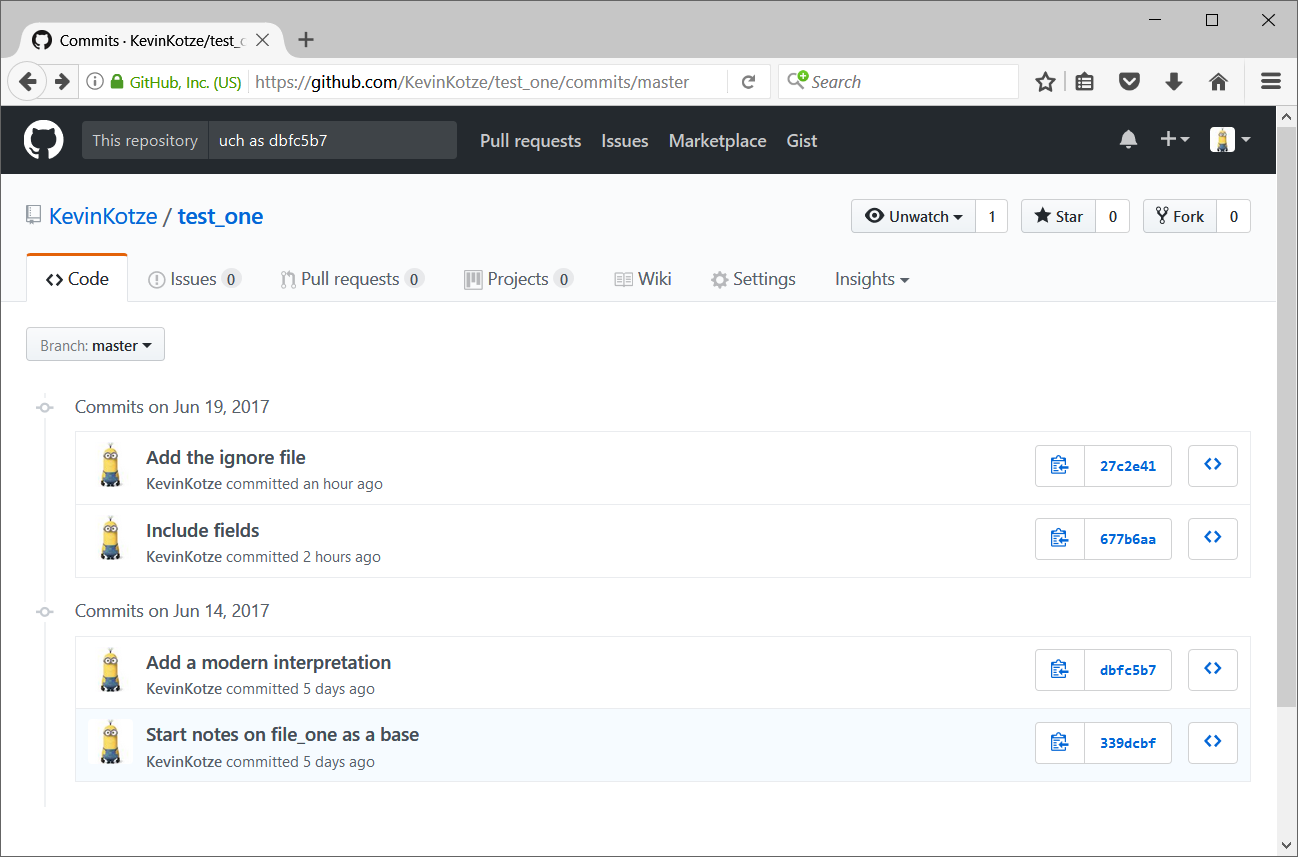The image depicts a screenshot of a GitHub website for a repository managed by "Kevin Kotz." The URL displayed is "github.com" and the organization name is "GitHub, Inc."

At the top, the repository is identified with a unique hash "UCH as DBFC at 5b7." Commit histories are prominently shown, detailing various updates made by Kevin Kotz.

1. **First Commit**:
   - **Date**: June 19th, 2017
   - **Description**: "Add the ignore file"
   - **Committer**: Kevin Kotz
   - **Time**: An hour ago

2. **Second Commit**:
   - **Action**: Includes fields
   - **Committer**: Kevin Kotz
   - **Time**: Two hours ago

Further down, more commit actions appear:

3. **Third Commit**:
   - **Date**: June 14th, 2017
   - **Description**: "Add a modern interpretation"
   - **Emoji**: Minion beside the commit message
   - **Committer**: Kevin Kotz
   - **Time**: Five days ago

4. **Fourth Commit**:
   - **Description**: "Start notes on file one as a base"
   - **Emoji**: Minion beside the commit message
   - **Committer**: Kevin Kotz
   - **Time**: Five days ago in the same section

The screenshot captures these detailed updates and highlights made by Kevin Kotz, with visual elements like emojis providing context and emphasis on specific commits.